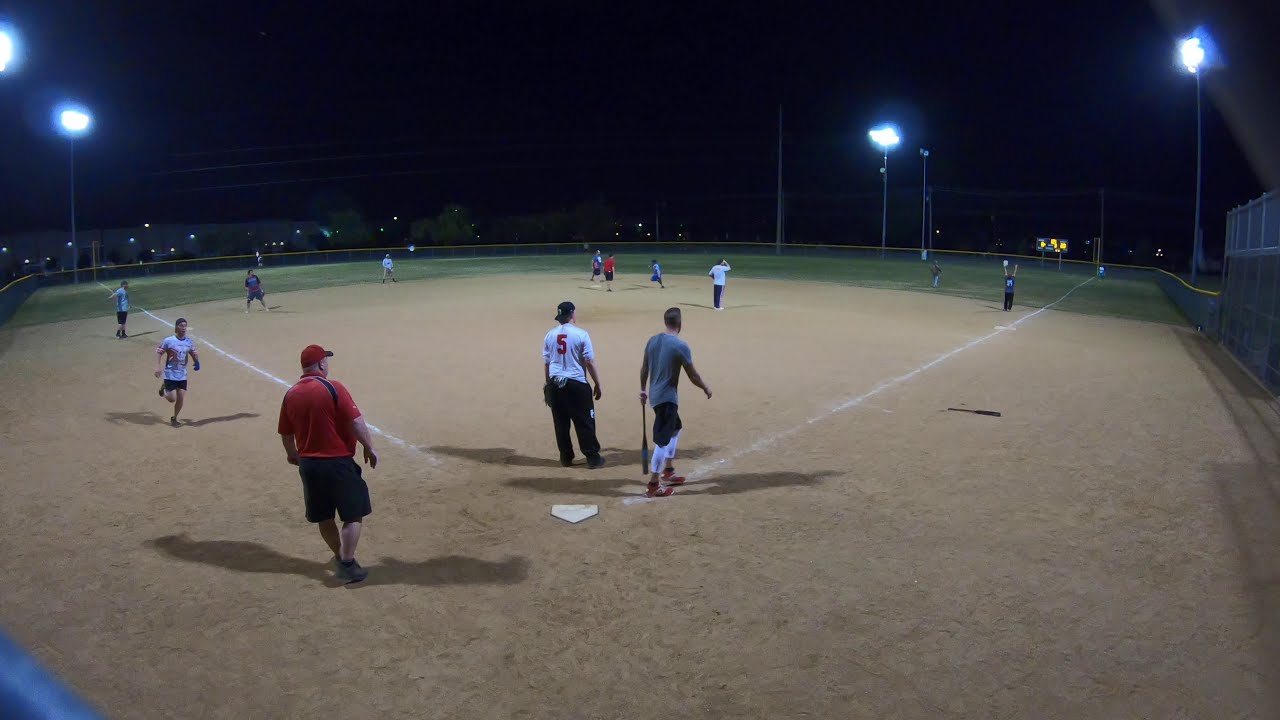This image captures an organized night-time baseball game in progress on an amateur field illuminated by several large lights. The scene is viewed from behind the diamond, showcasing the batter still holding his bat, likely having just hit the ball deep towards right field. The catcher, sporting a number five jersey, stands behind home plate, observing the ball's trajectory. An umpire, easily identifiable by his red shirt and dark shorts, is stationed behind the catcher. On the base paths, a runner is rounding third base heading home while another runner advances towards second base, suggesting that the batter may have hit a home run. The setting features a marked contrast with well-lit players and a darker background, emphasizing the focused intensity of the night game. The field transitions from a sandy diamond to grassy expanses beyond, giving the scene a quintessential amateur baseball ambiance.